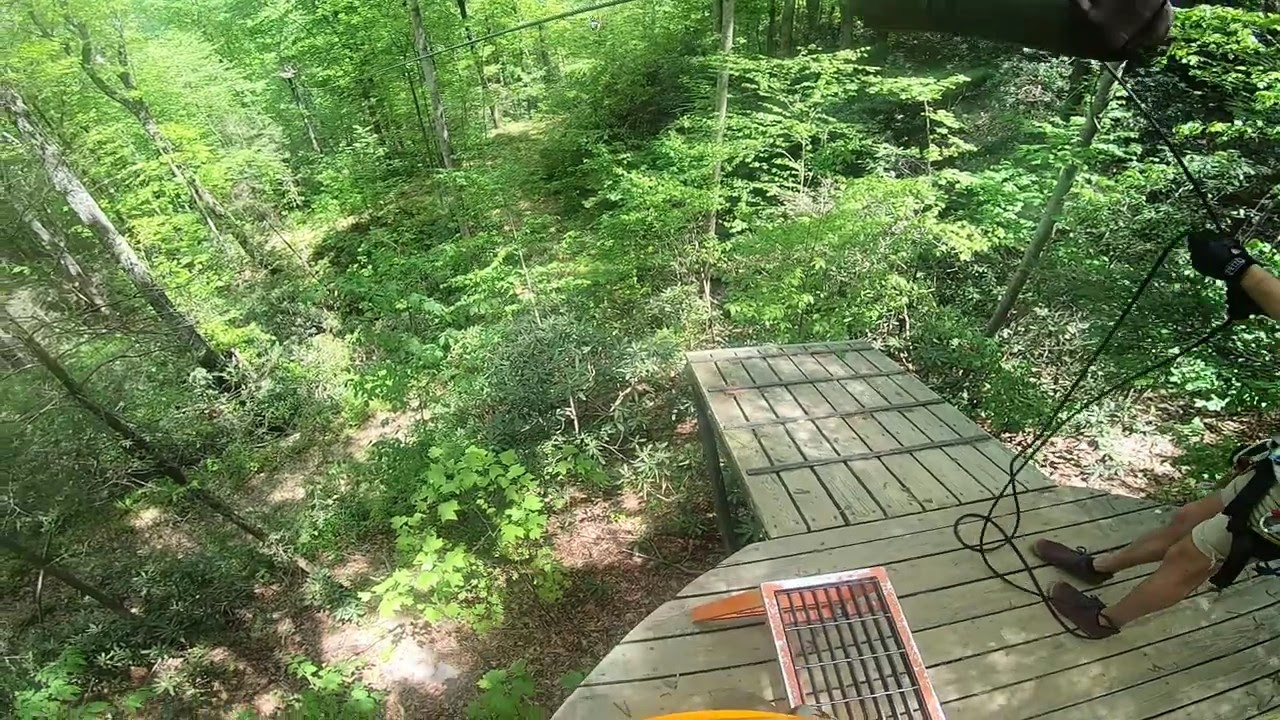The image is a high-angle color photograph in landscape orientation, capturing an outdoor scene dominated by lush greenery. In the foreground, there is a semi-circular wooden deck extending into a forested area. Attached to the semicircular deck is a plank walkway or pier that stretches outward, supported by poles at its far end. On the left side of the deck stands an orange table with yellow legs and a grid-like surface. On the right side of the image, a man wearing shorts, black sneakers, and heavy gloves is visible from the waist down. He is holding a black cable and a selfie stick, with a portion of a cell phone camera visible at the top of the stick. The cable appears to be connected to an object in the upper right corner of the frame, suggesting some form of setup for an outdoor activity, possibly bungee jumping or hang gliding. The surrounding area is densely populated with trees and foliage, emphasizing the natural, wooded environment.